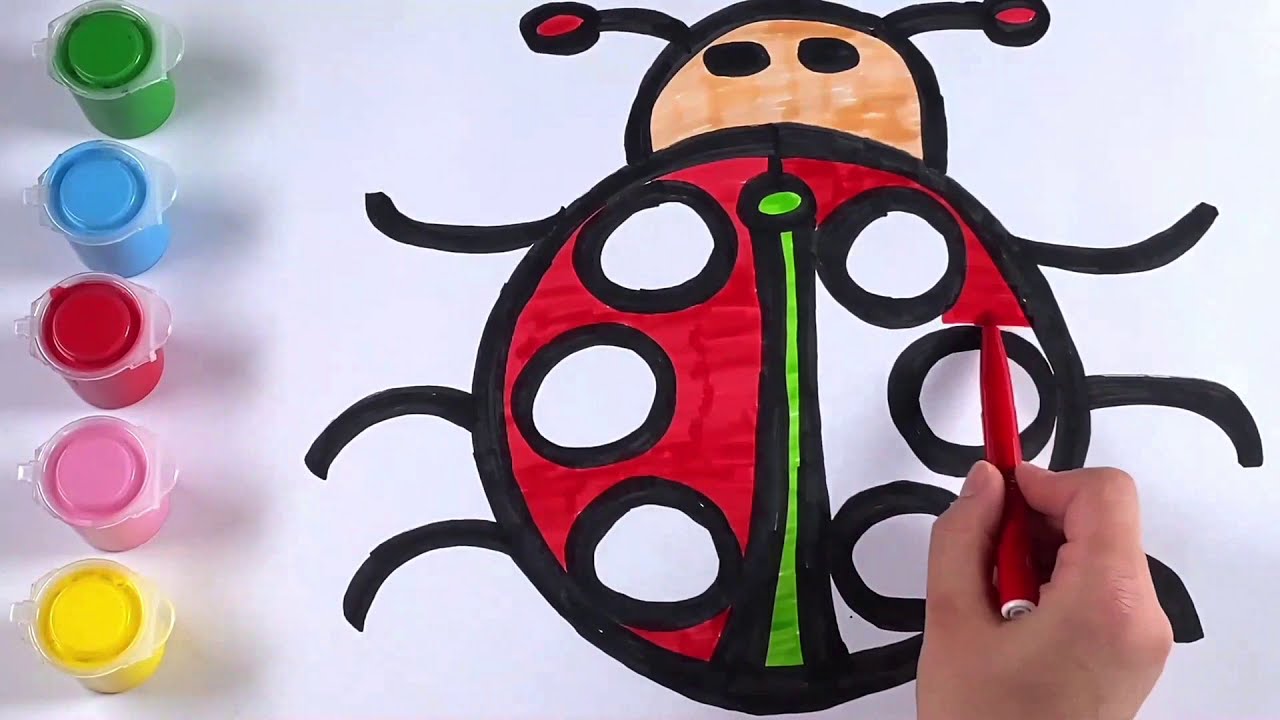This horizontal rectangular image captures a top-down view of a detailed drawing of a ladybug, being colored by what appears to be a child. On the left side of the image, five paint containers are aligned vertically in the colors green, blue, red, pink, and yellow, though the paints do not appear to be used on the drawing itself. The child’s hand, holding a red marker with a white top, is visible in the bottom right corner, actively shading the back of the ladybug in red.

The ladybug has a circular body with a light brown (or peach-colored) face, equipped with two black eyes devoid of pupils or additional design elements. Two antennae extend from the top of its head, each with a red circle at the tip. The back of the ladybug features several large, uncolored white circles outlined in black and a prominent vertical green strip running from the bottom up to the head area. Extending from the body are six black legs, positioning the ladybug in a classic top-down perspective. The image's background is a solid light gray, providing contrast to the vivid colors of the drawing.